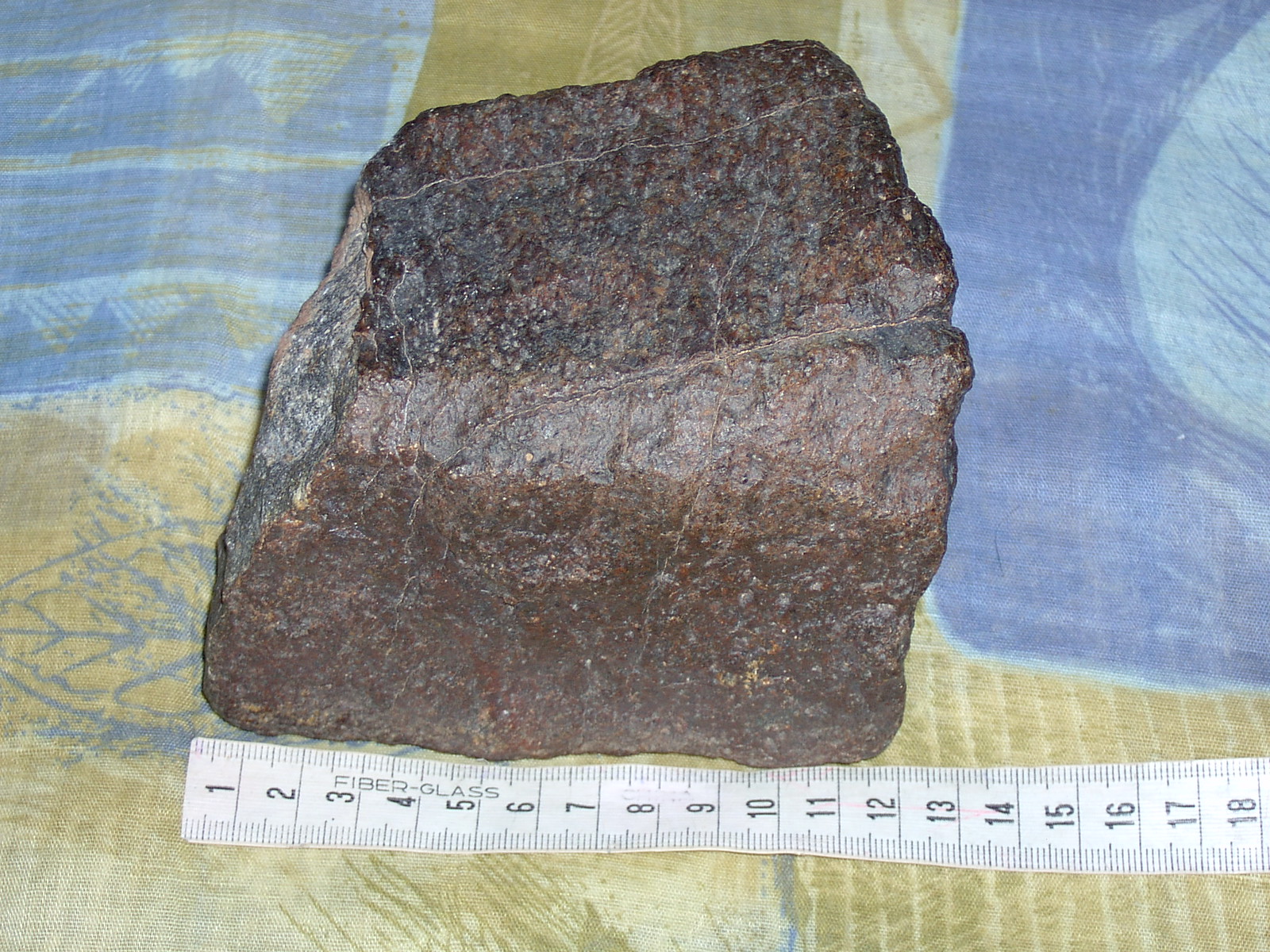This is a horizontally aligned rectangular sketch featuring a prominently placed rock specimen at the center. The rock has an intriguing shape, almost resembling a square with a triangular, mountain peak-like top. The rock's color transitions from dark brown with hints of gray at the top and bottom to a lighter brown and gray in the middle and on the sides. Specks of gray and white are scattered throughout its surface, adding texture.

Below the rock, a white tape measure is positioned to measure its width. The tape measure, which features black writing and is marked with "fiberglass," spans from the number 1 on the left to number 12 on the right, indicating that the rock is approximately 12 inches wide.

The background of the image is divided into two primary sections. The bottom portion is light brown with a few blue lines, suggesting a textured surface. The upper left and right sides of the background are predominantly blue. The left section of blue contains several horizontal streaks of light brown, while the right side features a half-circle of lighter blue, possibly resembling a decorative illustration of leaves or plants. Overall, the composition combines both detailed observation and artistic elements.